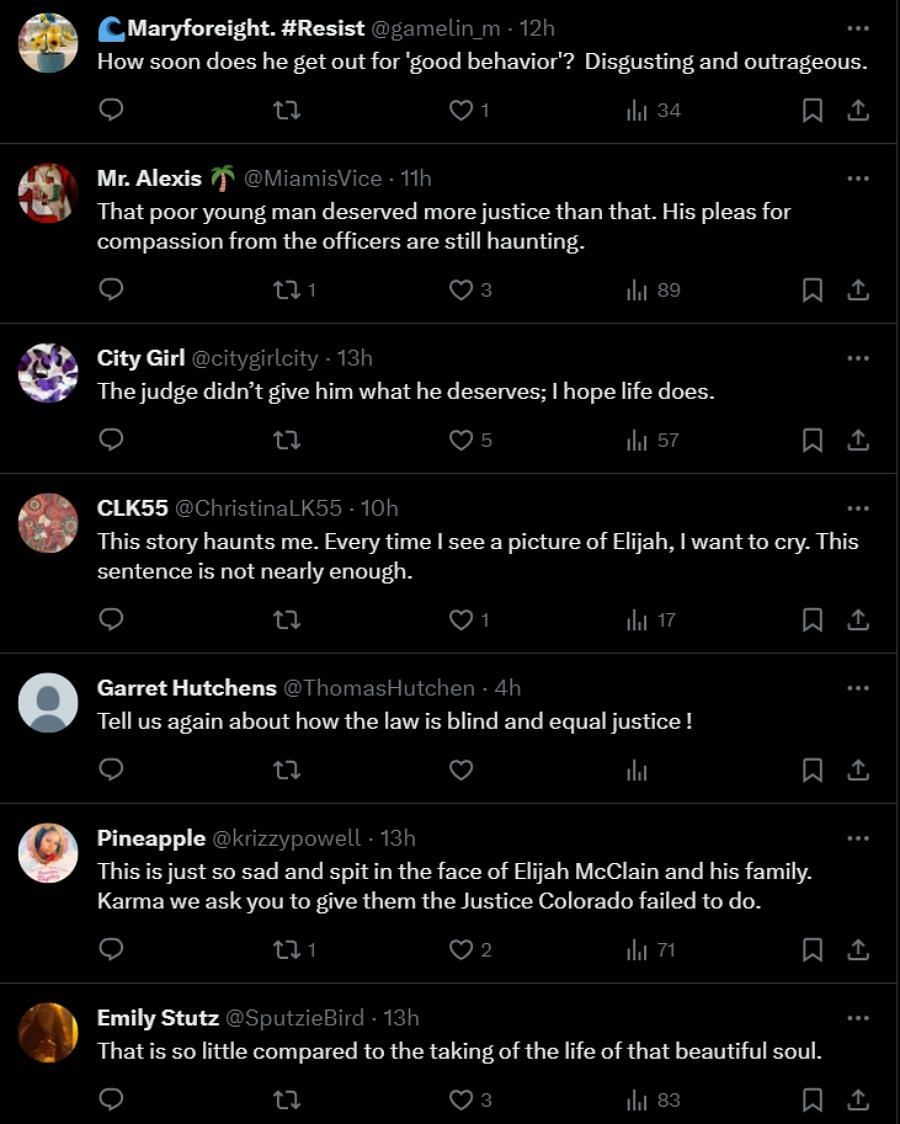This image captures a screenshot of a conversation on Twitter, displayed on a device that could be a computer, large tablet, or phone. The screen has a black background and shows a sequence of comments from several users discussing a controversial judicial outcome. 

Mary (@resist) expressed outrage with the comment, "How soon does he get out for good behavior? Disgusting and outrageous." Following her, Mr. Alex with a palm tree icon (@miamisvice) commented, "That poor young man deserved more justice than that. His pleas for compassion from the officers are still haunting." 

City Girl (@citygirlcity) added, "The judge didn't give him what he deserves. I hope life does," while CLK 55 (@ChristinaK55) expressed her distress, "This story haunts me every time I see a picture of Elijah. I want to cry. This sentence is not nearly enough."

Garrett Hutchins critiqued the justice system with, "Tell us again about how the law is blind and equal justice," and Pineapple commented, "This is so sad and a spit in the face of Elijah McClain and his family. Karma, we ask you to give them the justice Colorado failed to do."

Finally, Emily Stutz expressed skepticism about the comments’ validity, stating, "This is so little compared to the taking of the life of that beautiful soul. Once again, we have people commenting about things they probably have absolutely no knowledge of. That's people today. They can post anything they want to without knowing a thing."

The overall sentiment in the conversation is one of frustration and sorrow, particularly in response to the judicial handling of Elijah McClain's case.